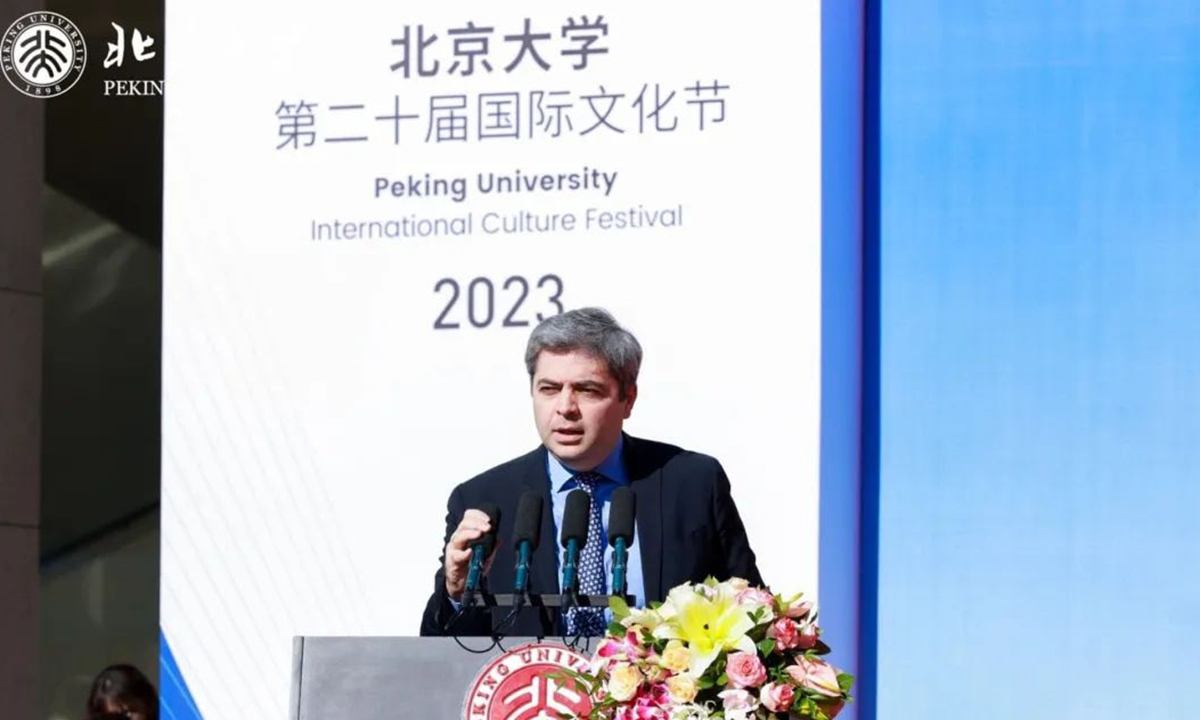In the image, a middle-aged man in a dark navy suit, light blue shirt, and navy white polka dot tie is standing at a gray podium adorned with a bouquet of yellow lilies, pink, and white roses. The podium features a white seal with red letters that read "Peking University." He is speaking into four microphones. Behind him, a large banner reads "Peking University International Culture Festival 2023" in black English letters, with additional Japanese text above against a white backdrop. To his side, a woman with black hair and a white face sits looking down at her lap. The setting is predominantly indoors, divided with blue hues to the right and black to the left. The emblem of Peking University also appears on the banner, reinforcing the university's prominent focus in the event.